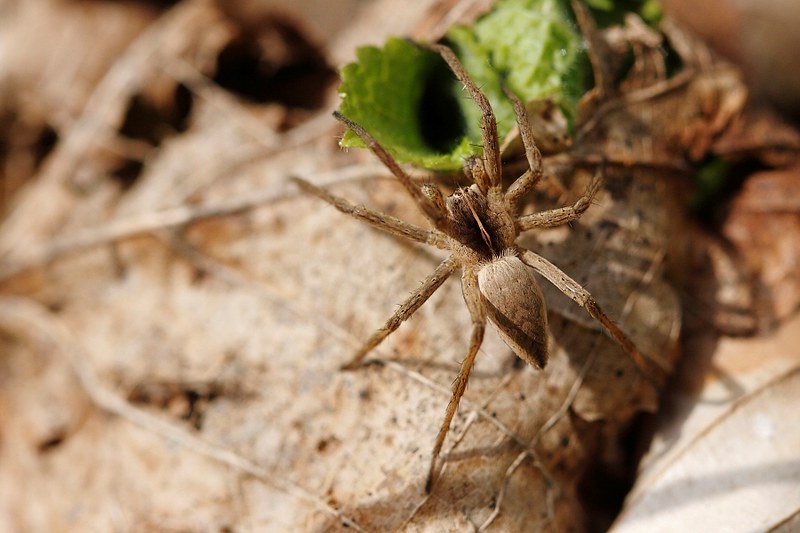This is a close-up, full-color photograph taken outdoors during the day, showcasing a large brown spider intricately camouflaged against a backdrop of dead leaves and scattered vegetation. The spider, with its blend of light and dark brown hues and fur on its legs and abdomen, expertly blends into the environment. Its body, described as a teardrop or triangular shape, features a dark black top with a distinguishing lighter brown stripe running through it, and its posterior is almost white. The ground is strewn with dead, brown leaves, twigs, and rocks, with one strikingly green, cylindrical leaf positioned prominently in the upper center of the composition. The spider's front legs are extended, grasping this singular vibrant leaf, contrasting sharply with the otherwise lifeless surroundings.